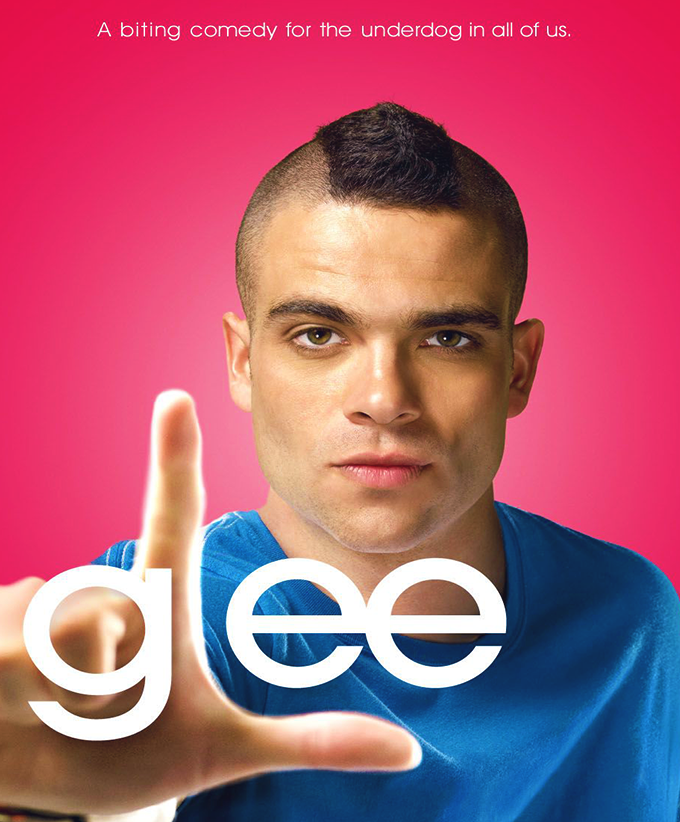This full-color promotional photograph features a single young man named Puck, one of the characters on a show, against a pink background. The text at the very top, in bold white letters, reads, "A biting comedy for the underdog in all of us." Puck, with dark hair, brown eyes, and a short mohawk strip down the center of his otherwise shaved head, is positioned centrally, reminiscent of a headshot. He is wearing a blue short-sleeved shirt and has his hand prominently in the foreground, making the "L" loser symbol. This "L" integrates with the white letters "G-E-E" at the bottom of the image to spell out "G-L-E-E."